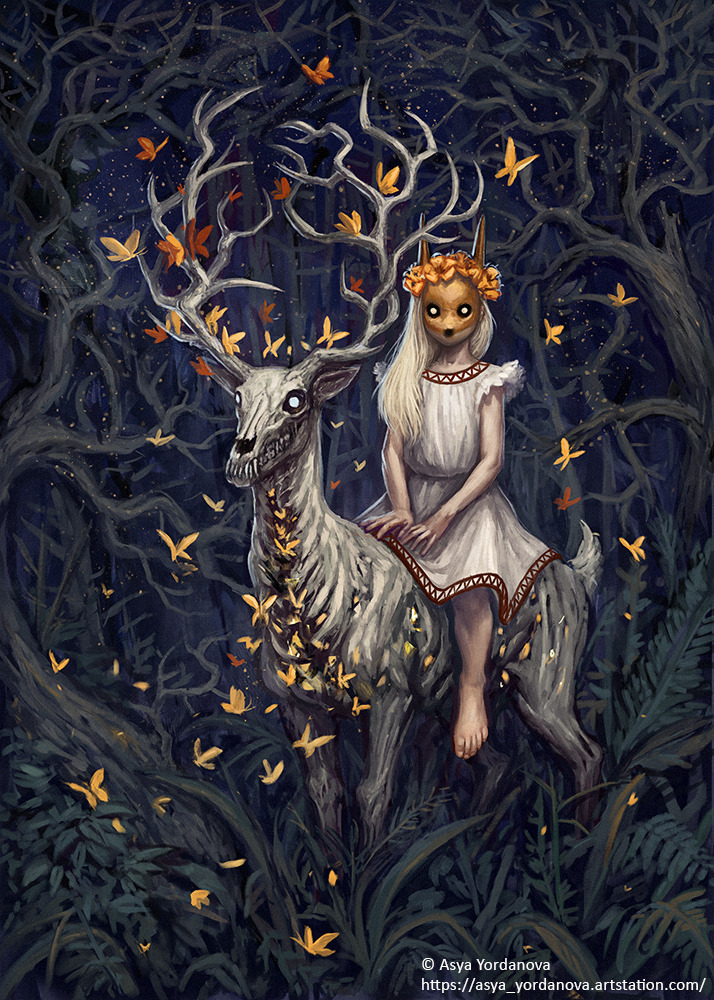The image depicts a dark fantasy scene reminiscent of "The Nightmare Before Christmas." A ghostly girl with long, white hair crowned with flowers and glowing eyes rides bare-footed on a fantastical stag. Both the girl and the stag have a macabre, lifeless appearance, with the girl's skin eerily pale and her lips unnaturally pursed, resembling a dead doll. She wears a flowing white dress that adds to her spectral look. The stag, sleek and silvery with metallic undertones, has haunting glowing eyes and a face marked with stitches across its nose, contributing to its eerie visage. The immense antlers of the stag are adorned with birds, while butterflies flit around them, some perching delicately on the antlers. The background features an ominous forest of twisted, black trees, punctuated by dark green ferns and leaves at the bottom of the image. The atmosphere is chilling and otherworldly, with vibrant butterflies in hues of yellow, red, and orange providing a striking contrast to the dark, surreal landscape. A copyright mark in the bottom right corner credits the artist, ASYA Yordanova.